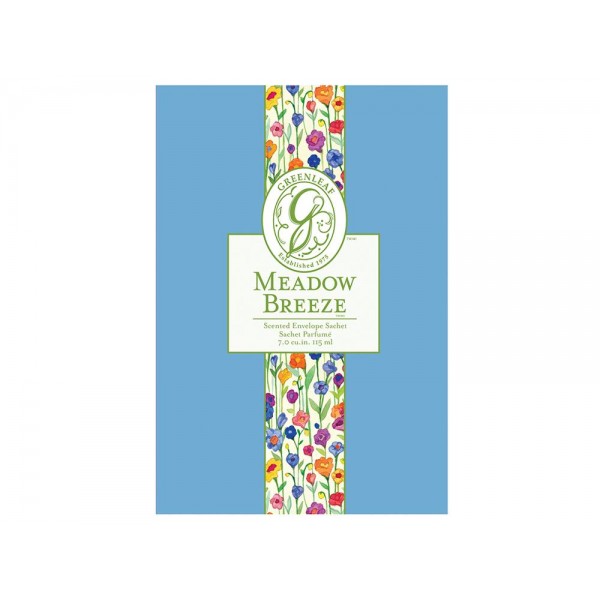This digital image showcases the cover of a scented envelope product called Meadow Breeze by Greenleaf, a company established in 1973. The center of the image features a prominent circular logo with a stylized "G" in green, surrounded by green text that reads "Greenleaf Established 1973". Below this logo, additional green text within a white, green-bordered box states "Meadow Breeze scented envelope sachet, sachet perfume 7.0 cu.in. 115ml". The background of the image is light blue on both the left and right sides, with a vibrant vertical strip of multicolored flowers, including shades of blue, purple, red, orange, and yellow, adorned with green stems and occasional green leaves running down the center. The white label in the middle partially overlaps the floral design, adding a clean and visually appealing element to the composition.